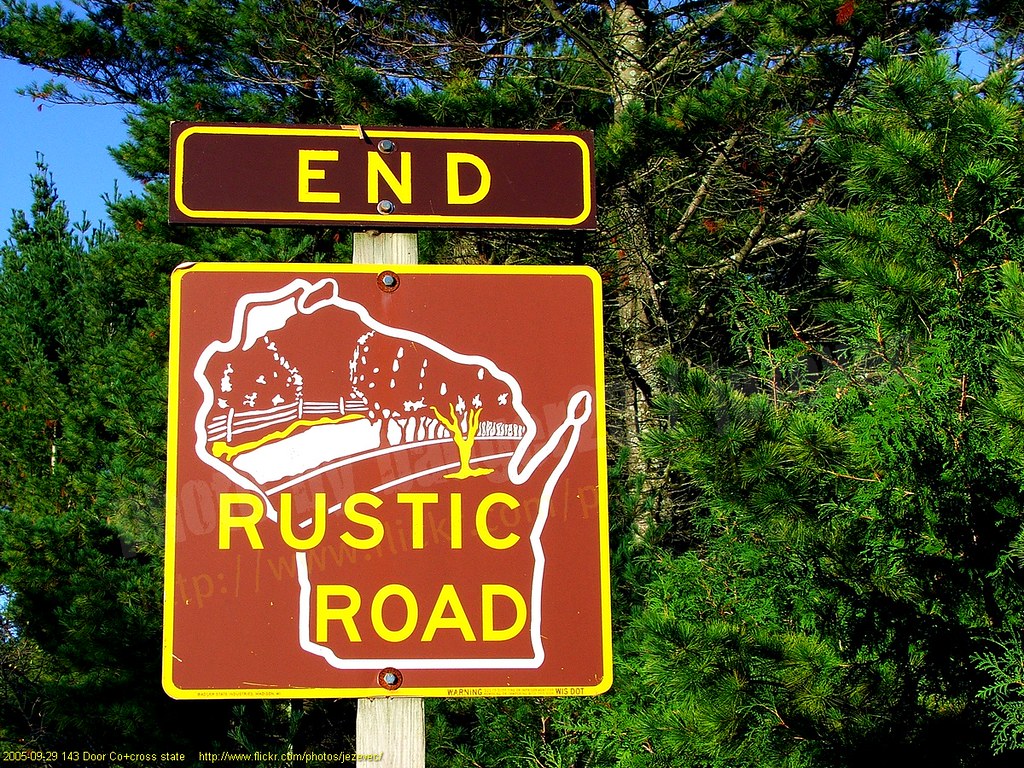The image captures a scenic, outdoor setting dominated by a massive tree with a thick trunk and numerous sprawling branches that take up most of the frame. The tree's dense foliage obscures parts of the sky, though patches of vibrant blue peek through the canopy. In front of this natural backdrop stands a prominent road sign split into two sections: the top sign reads "End" in yellow on a brown background, while the bottom sign is red with a yellow border and declares "Rustic Road," featuring an illustration of a tree-lined road and a fence. A small watermark in the bottom left corner indicates the photo was taken on September 29, 2005, and includes some specific location or web address details. The overall scene exudes a sense of tranquility and picturesque charm.